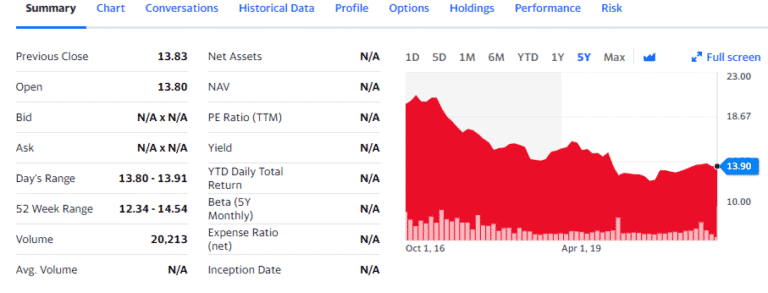This screenshot captures a detailed view of a stock menu interface. At the very top, the section labeled "Summary" is highlighted in black, indicating that this is the current screen being viewed. Surrounding this are other navigational links in blue text, including "Chart," "Conversations," "Historical Data," "Profile," "Options," "Holdings," "Performance," and "Risk."

Beneath this menu is a pale gray line dividing the navigational panel from the main data display area. The left side of this area contains key financial metrics presented in black text across two rows. These metrics include:

- **Previous Close:** 13.83
- **Opening Price:** 13.80
- **Bid:** N.A. × N.A.
- **Ask:** N.A. × N.A.
- **Day's Range:** 13.80 to 13.91
- **52 Week Range:** 12.34 to 14.54
- **Volume:** 20,213
- **Average Volume:** N.A.
- **Net Assets:** Not available
- **N.A.V.:** Not available
- **P.E. Ratio (TTM):** Not available
- **Yield:** Not available
- **Year-to-date Daily Total Return:** Not available
- **Beta (5-Year Monthly):** Not available
- **Expense Ratio (Net):** Not available
- **Inception Date:** Not available

Important numerical values are highlighted in bold for emphasis. 

To the right of this data, a graph is present to visually represent the stock's price movements. This graph offers multiple time frame options such as one day, five days, one minute, six minutes, year-to-date, one-year, five-year, and max. Additionally, there is an option to view the graph in full screen.

The graph displays the fluctuations of the stock price over a specific period, from October 1st, 2016, to April 1st, 2019.